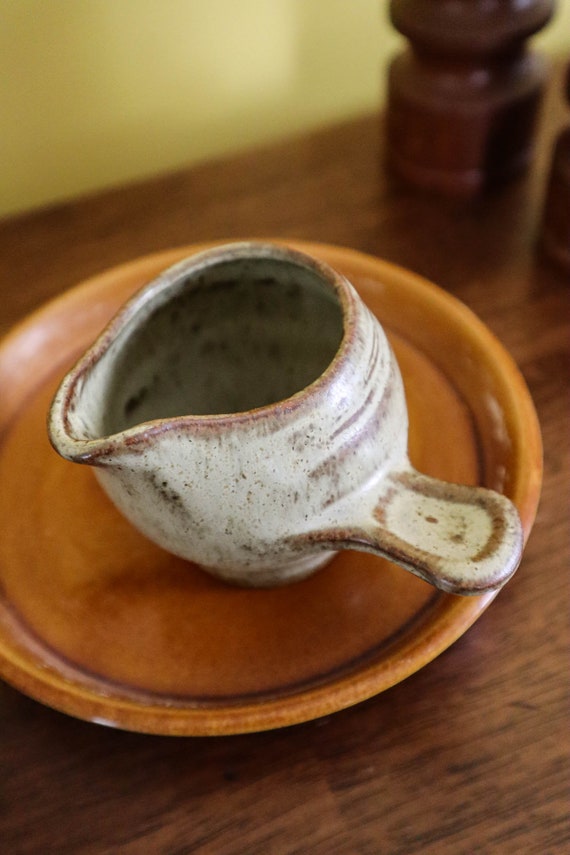This detailed photograph showcases a rustic scene centered on a dark wooden table or countertop, which serves as the backdrop. The focal point of the image is a small, light orange ceramic saucer with a notable raised lip around the edge. Seated on this saucer is an intriguing ceramic pouring utensil that exudes an aged charm. The utensil is predominantly white with brownish markings near the handle and the spout, which is funnel-shaped for easy pouring. The design of the handle is unique, reminiscent of a short, straight piece rather than a traditional curved handle. The interior of the cup is hollow and dark, shadowed by its shape. Surrounding these central items, the background reveals a glimpse of some wooden shakers, likely salt or pepper, against a light yellow wall, adding to the overall artsy and earthy aesthetic of the photo.